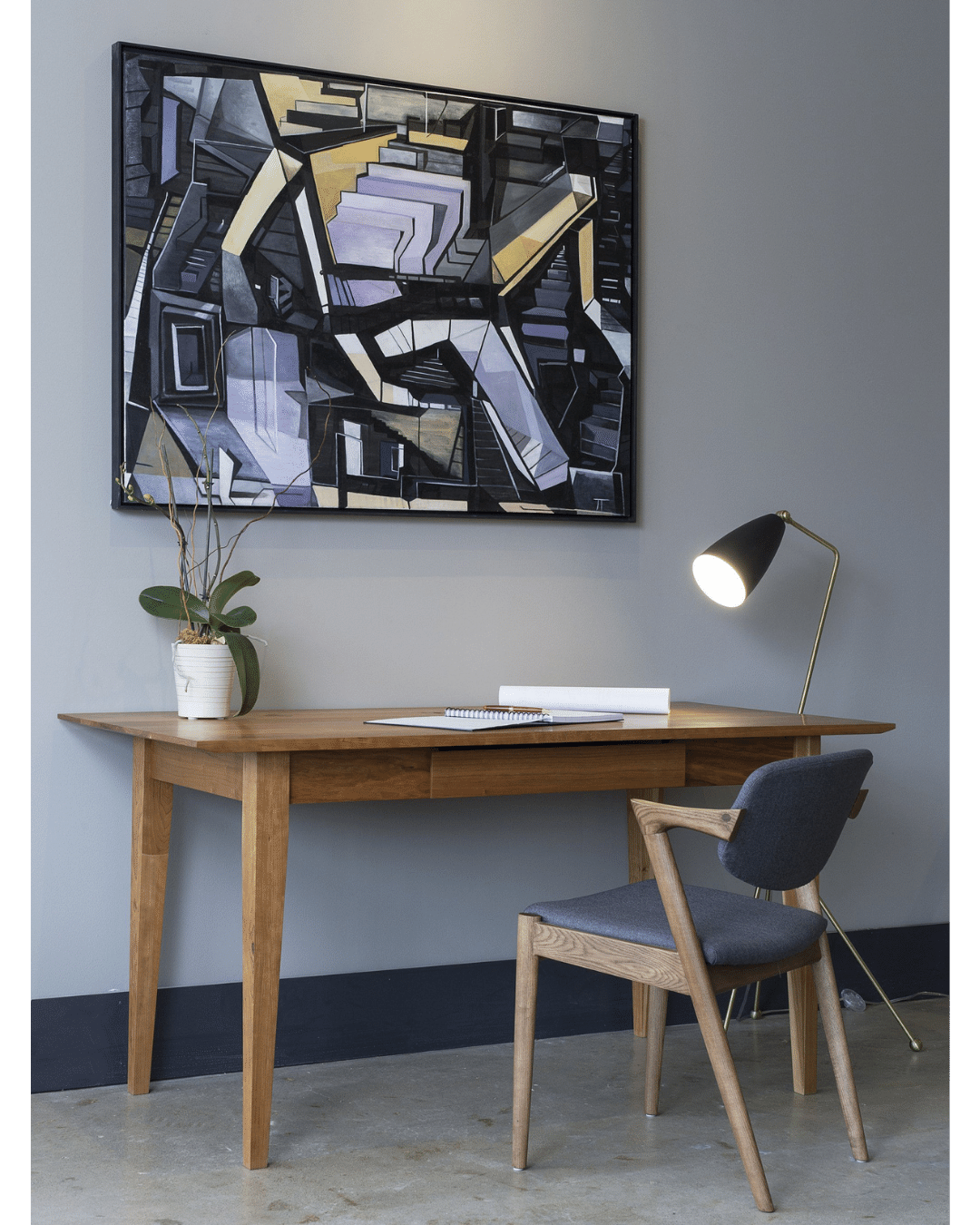The photo captures a minimalist office setting, characterized by a small brown desk with a partially pulled-away chair that features a blue cushion on the seat and back, and brown wooden armrests and legs. An open notebook with a pen resting on top and a separate piece of paper are situated near the center of the desk. A small floor lamp, extending slightly past the table and bent towards it, illuminates the workspace. In the upper left corner of the desk, there is a white planter with a slightly dying plant. Above the desk, hanging on the gray wall, is a large, contemporary piece of abstract art that combines angular shapes in light purple, dark purple, black, gray, yellow, and orange hues, with bold lines and swirls, set within a large frame. Everything rests on a beige floor, contributing to the overall subdued gray and neutral tones of the room.